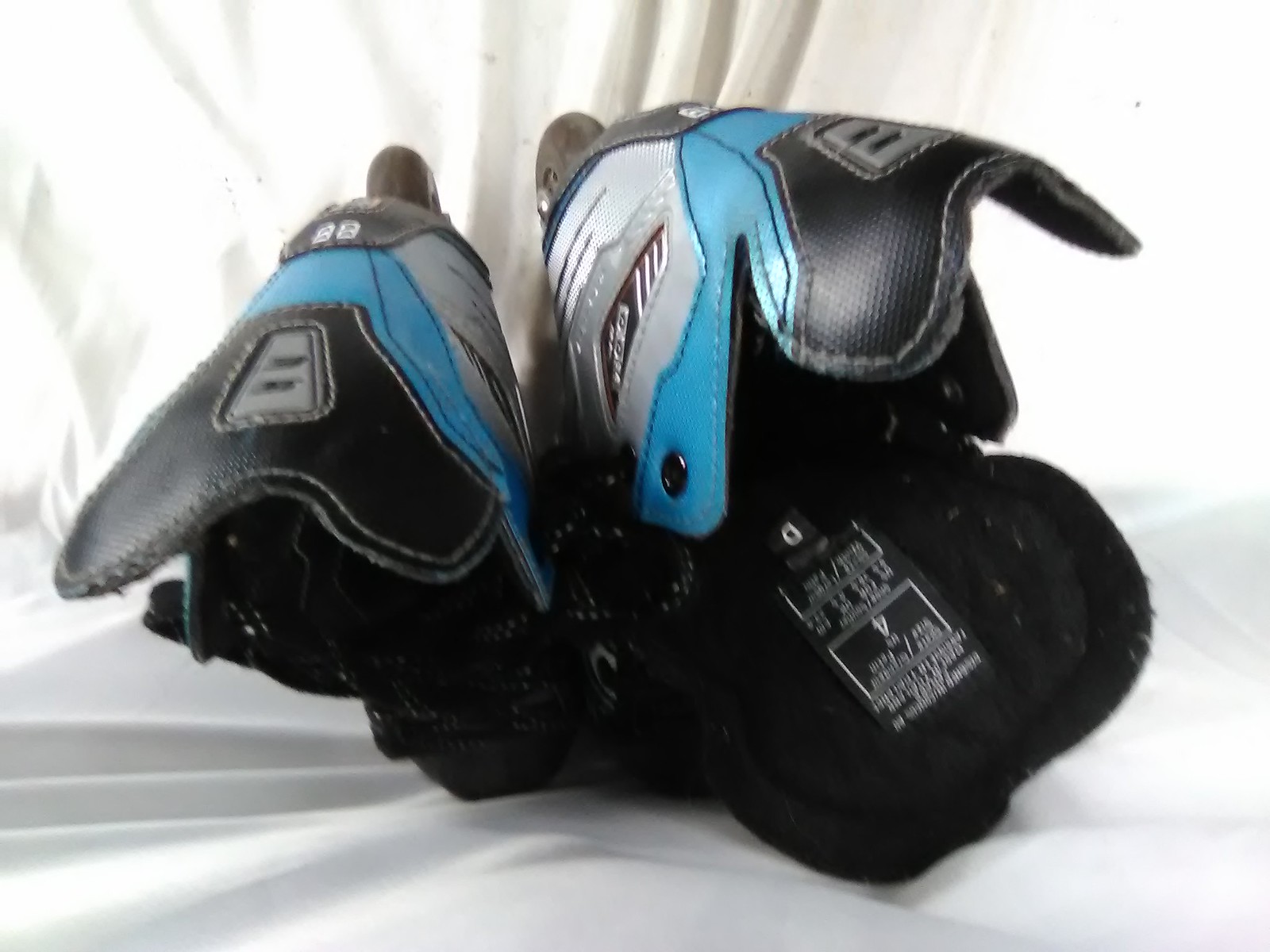This slightly blurry, sunlit photo captures a pair of rollerblades resting upside down on a wrinkled white fabric surface, with their laces touching the cloth. The rollerblades are positioned parallel to each other, with the collars facing the camera and the toes pointing downwards. The boots feature a black, gray, silver, and light blue exterior, with black grommets for the laces and black wheels protruding at the top of the image. The inside of the boots, including the tongues, are black and some fuzz is visible. A black tag inside displays a size of 4D. The background is dominated by a softly pleated white curtain, bathed in bright sunlight.